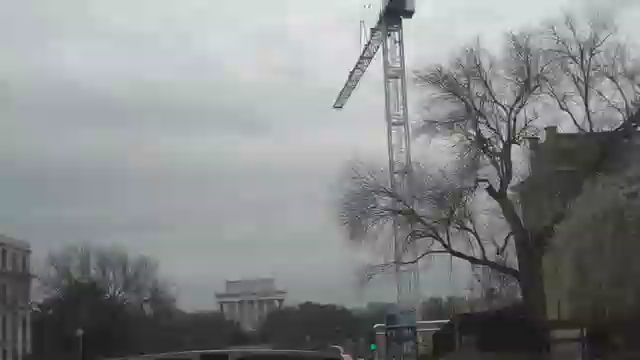This color photograph, taken outdoors on an overcast and almost foggy day, captures the moody ambiance of a very cloudy sky that dominates most of the image. In the distant background, a faint silhouette of a structure that resembles the Lincoln Memorial emerges through the haze, adding a layer of historical significance to the scene. Flanking the sides of the composition are trees; the one to the left is bare, suggesting the winter or late fall season. Meanwhile, to the right, the edge of a large stone building comes into view, its presence suggesting a setting within an urban or historically rich area.